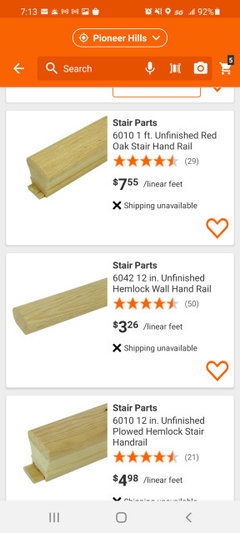This image is a detailed screenshot captured from a mobile device's display, showcasing a shopping website interface. The status bar along the top is populated with numerous icons typical of such devices, including indicators for time, new mail, an alarm clock, location services, data signal strength, battery status, and more.

Central to the screenshot is the website's header, which features an orange background. Within this section, there is a rounded rectangular location selector currently set to "Pioneer Hills," marked by a location icon and a drop-down arrow for changing the location. Below this header is an empty search bar, inviting users to search for items on the site. To the right of the search bar is a shopping cart icon with a numeric indicator "5" above it, suggesting there are five items currently in the user's cart.

The main content area of the screenshot displays three distinct products, each presumably related to wooden stair parts. Each product listing includes an image, a detailed description, customer reviews, pricing information, and an availability status indicating whether the items are in stock.